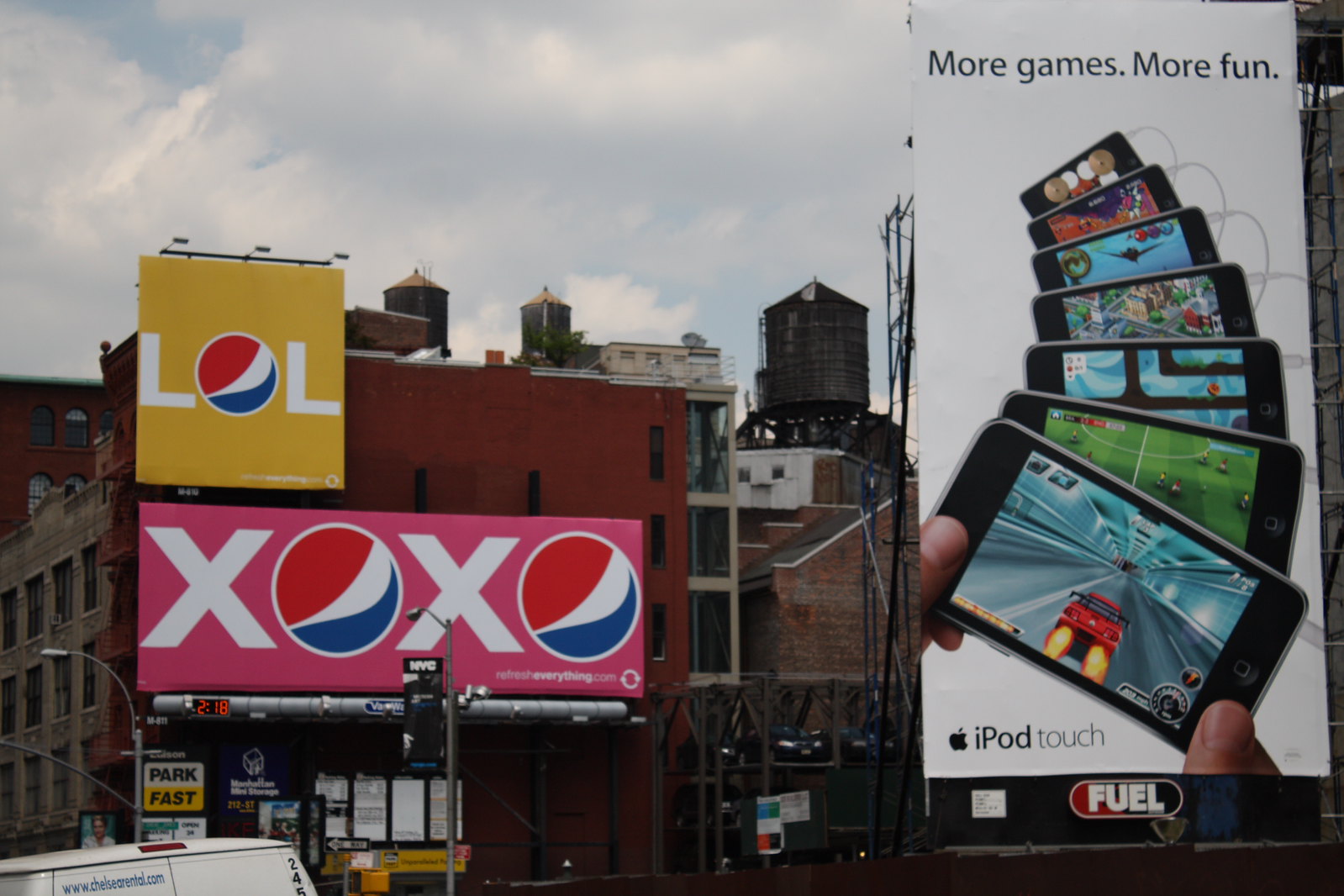This color photograph captures a bustling urban street scene during the daytime. Dominating the right side of the image is a vertical billboard advertising the iPod Touch. The ad features seven different iPods, all angled and lined up, each connected by white cords. The devices are displayed against a white background, with the tagline "More games, more fun" above them. Each iPod showcases a different game, emphasizing the device's gaming capabilities. At the bottom of this billboard is a red and black oblong icon with the word "Fuel" in white letters.

To the left, in the distance, are two stacked billboards mounted on the side of an older brick building. The lower billboard shows "XOXO" in large white letters, with the O's replaced by Pepsi logos, all set against a pink background. Above it, the smaller billboard displays "LOL," with the central O again replaced by the Pepsi logo, in white letters on a pink background.

The brick building itself is a multi-story structure with red bricks and a beige facade facing the street, featuring darkened windows. Off in the distance, there's a view of water towers rising above other buildings, under a cloudy sky. In the foreground, partially visible, is a parked van, adding to the urban atmosphere of the scene.